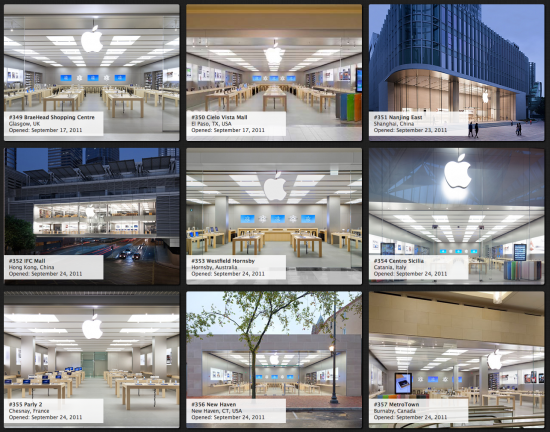This image features a collage of nine live camera feeds from various Apple store locations around the world, each housed within a separate square making up a three-by-three grid. 

**Top Row:**
1. **Upper Left**: Displays an Apple store at an undisclosed shopping center in Glasgow, UK. The address is partially blurred, but it's noted that the store opened on September 17, 2011. Various kiosks, likely showcasing cell phones, are visible, along with a backdrop featuring two blue elements.
   
2. **Upper Middle**: Captures the Apple store at Cielo Vista Mall in El Paso, Texas. The store layout appears organized with sections dedicated to different Apple products.

3. **Upper Right**: Shows an Apple store location in Shanghai, China, featuring a sleek interior design typical of Apple retail environments.

**Middle Row:**
1. **Middle Left**: Represents an Apple store in Hong Kong, China. This store, like others in the grid, opened on September 24, 2011, and features an array of product displays.

2. **Middle Center**: Features an Apple store in Australia, continuing the uniform design aesthetic of Apple stores worldwide. This particular location also opened on September 24, 2011.

3. **Middle Right**: Depicts an Apple store in Italy, with an organized interior showcasing the same opening date as its counterparts in the middle row.

**Bottom Row:**
1. **Bottom Left**: Location and details are not specified, but it follows the same format, showing live footage with the store's unique address in the bottom left-hand corner.
   
2. **Bottom Middle**: Similar to the others, it shows an Apple store with live feed, address, and retail layout.

3. **Bottom Right**: Continues the theme of live camera footage showcasing another Apple store location, complete with address and opening information.

All stores featured in this collage share the hallmark Apple retail design with clean lines, product-focused displays, and the iconic Apple logo. Specific dates of opening in September 2011 are noted, emphasizing the consistency of new store launches during that period.